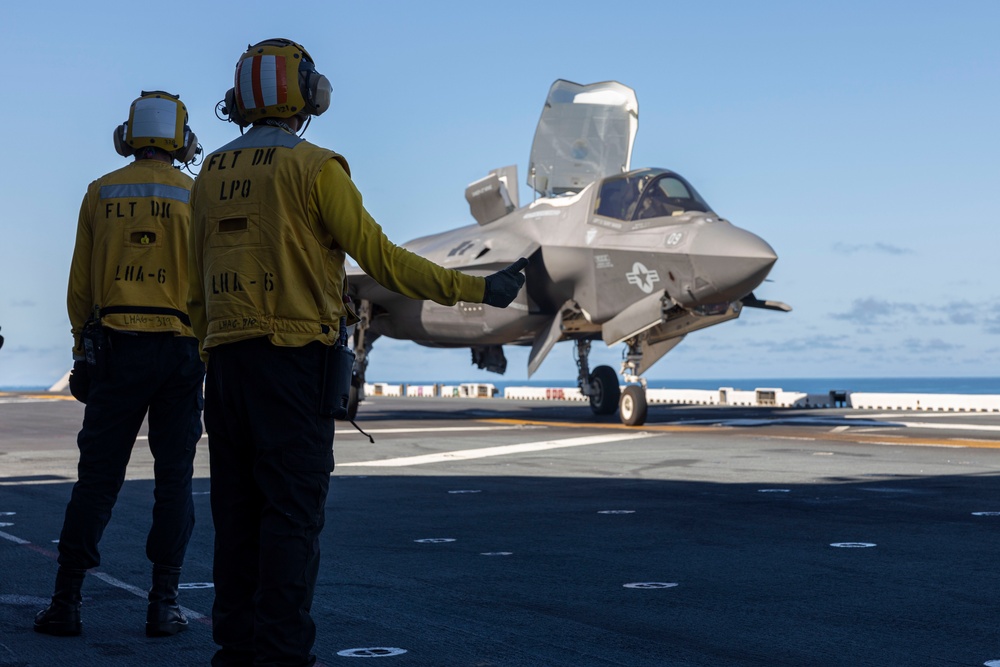This detailed photograph captures two gentlemen standing on the runway of an aircraft carrier, overlooking a small gray fighter jet, likely a military plane, which features a gray star emblem near its small front window. The background showcases the horizon with blue sky and ocean, hinting at the vessel's location. Both men, seen from behind, are equipped with yellow safety helmets adorned with white stripes, noise-canceling headphones, and long-sleeved yellow safety jackets with black pants. Their jackets prominently display the stencil text "FLY on LPD," accompanied by additional stenciled markings that are difficult to decipher, possibly reading "F.L.T.," "D.K.," "L.H.A.6-319," or similar variants. One man, differentiated by his black gloves, is giving a thumbs-up, suggesting readiness for the jet, which has its top hatch open and wheels down, indicating imminent takeoff or arrival.